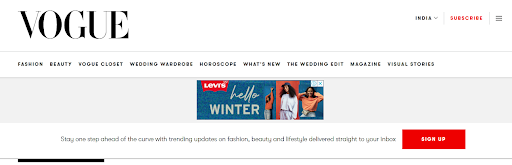The image is a screenshot of the Vogue website, featuring the iconic Vogue logo prominently displayed at the top left corner in black. The menu bar beneath the logo includes various subcategories: Fashion, Beauty, Vogue Closet, Wedding Wardrobe, Horoscope, What's New, The Wedding Edit, Magazine, and Visual Stories. The text for the last subcategory is too small to read clearly.